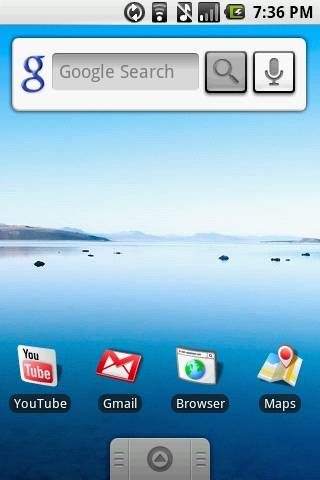This is a screenshot of what appears to be an old-fashioned scheduling or reader gadget. At the top, there are several symbols: an Internet icon, a volume icon which resembles a music symbol, another Internet icon, and a battery indicator. The time displayed is 7:36 PM. Below these symbols lies a white bar with a dark medium blue border featuring a lowercase "g" for Google on the left. Adjacent to this is a light gray search bar labeled "Google search," accompanied by two icons on the right—a magnifying glass (search button) and a volume button.

The background of the interface displays an image of a serene natural landscape. A blue sky spans across the top, with a small, low mountain range in the distance. In the foreground, there's a body of water—either a lake or an ocean—with visible rocks scattered across its surface.

At the bottom of the screen are four app icons with their labels:
1. **YouTube**: A white square logo with the word "Tube" in white against a red background.
2. **Gmail**: An envelope icon with red outlines.
3. **Browser**: A white square background featuring a search bar and a globe icon.
4. **Maps**: A folded map icon with a red pinpoint.

Below these app icons, centered at the bottom of the screen, is a gray square with three horizontal lines on the left and right sides. In the middle of this square is a circle containing a triangle pointing upwards.